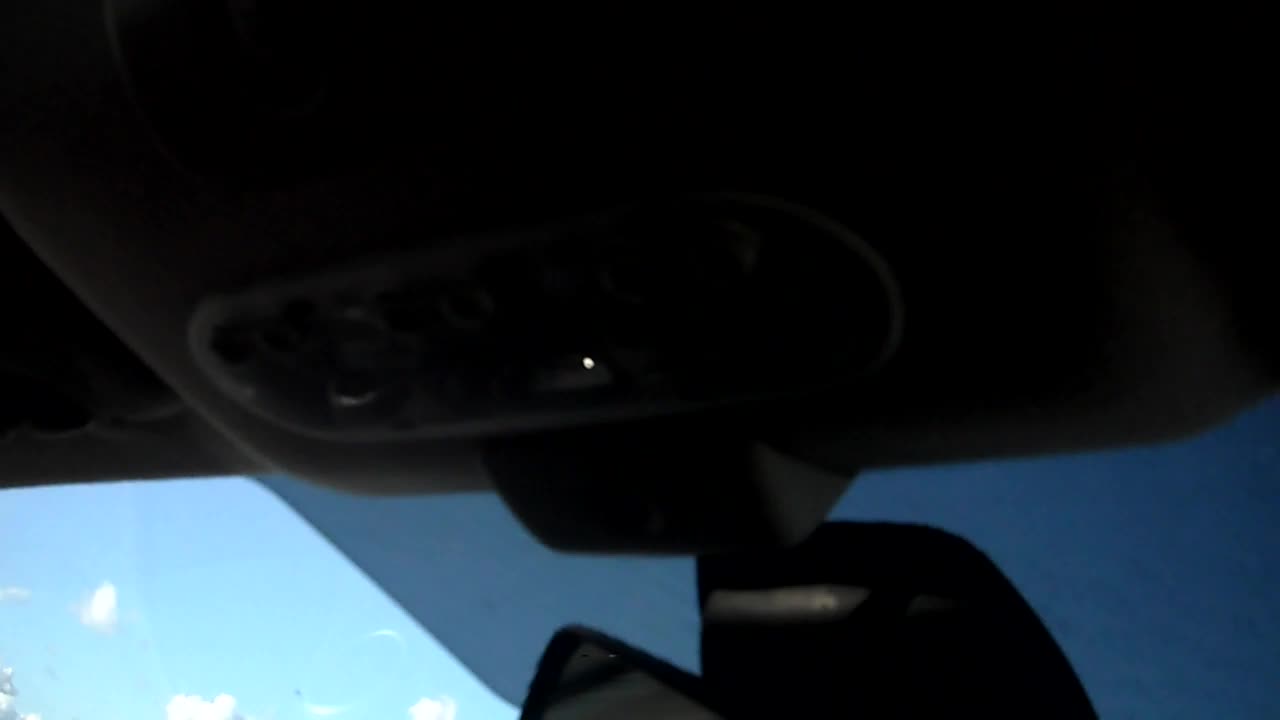This photograph, taken from the interior of a black car, focuses on the front windshield and surrounding areas. The interior features black elements, including a small mirror and sections around the windshield, along with an overhead console for storing sunglasses. The sky visible through the windshield is blue with scattered white clouds, suggesting it's daytime. Distinctly, the left side of the windshield is brightly illuminated by sunlight, while the right side appears to have a piece of plastic or window tint overlay. This overlay transitions from light blue to dark blue, obscuring the clouds and featuring small dimples, possibly indicating a test for window tint. The image is somewhat blurry and lacks a specific focal point, potentially suggesting it was taken accidentally. The shot hints at the ceiling and upper console of the car, with some elements that might be confused with the back section, such as where a station wagon's or minivan's brake light housing would be located, but the primary focus remains on the front windshield area.